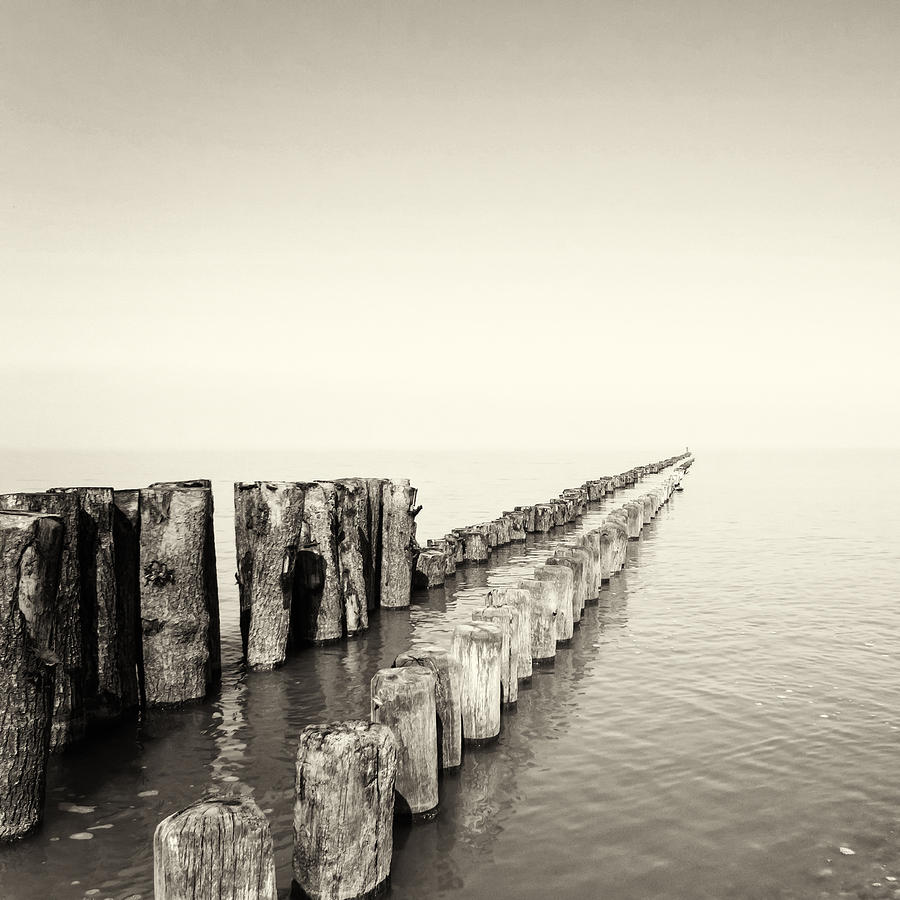A serene, artistic black-and-white photograph captures a scene of calm water, likely a bay, with a hazy sky becoming progressively lighter towards the horizon. In the foreground, two parallel rows of weathered wooden posts emerge from the water, appearing as remnants of an old fishing pier or perhaps wave-breaking structures. The posts on the right are uniformly white with black specks, while those on the left are slightly taller at first before matching the right row's height, appearing a bit darker. The water between and around the rows is notably darker, suggestive of shadows cast by the posts. Scattered bubbles float in the bottom right corner. The scene, devoid of text, evokes a sense of timelessness and tranquility, characteristic of an old photograph or a detailed pencil drawing. The stillness of the water and the artful composition hint at a secluded, protected shore.